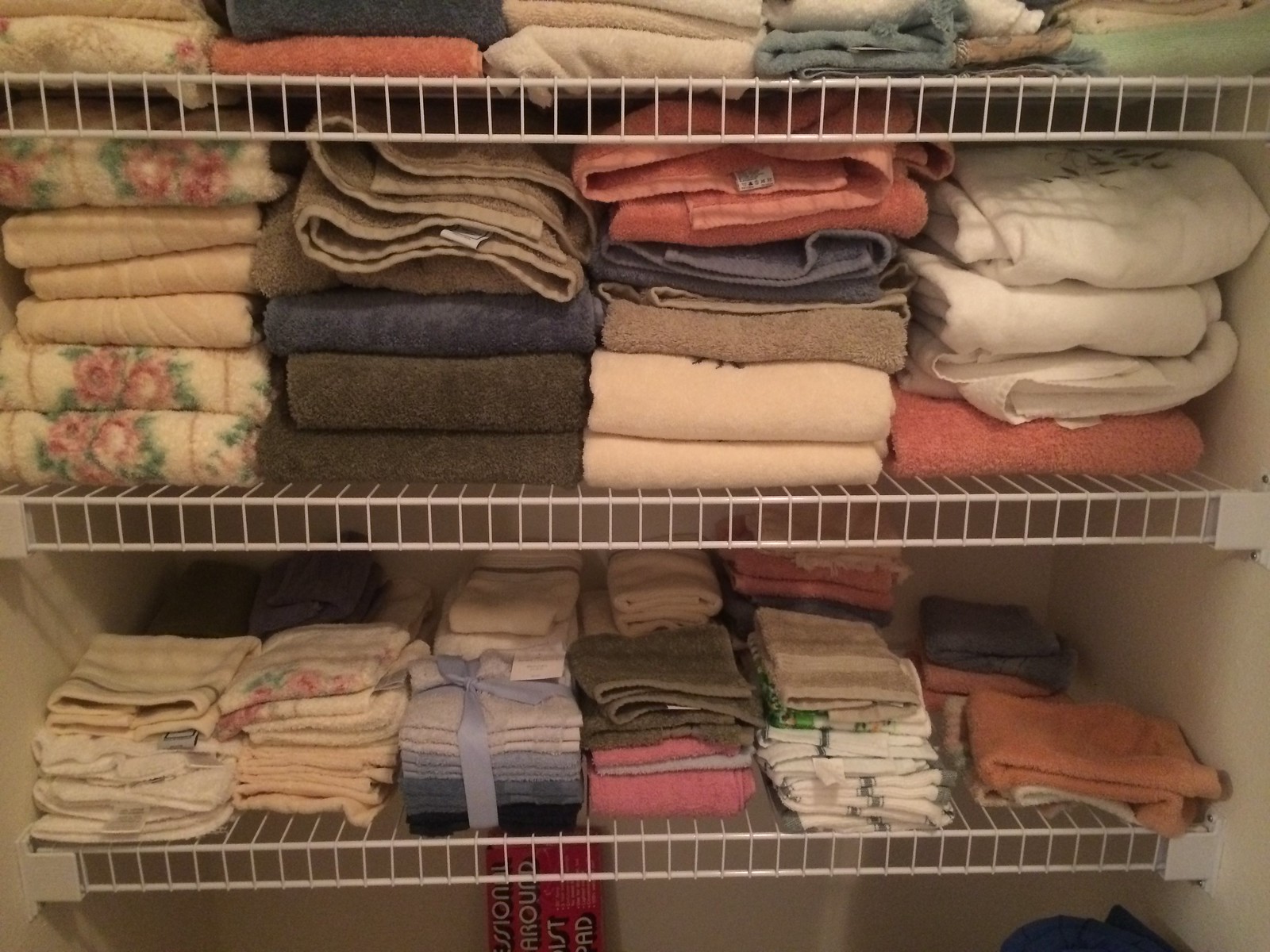This photograph captures a neatly organized linen closet, seemingly in a home, showcasing three white wire shelves against white walls. The bottom shelf features an array of neatly folded washcloths and hand towels in various colors including brown, white, pink, and blue, along with a bundle of brand new washcloths tied with a blue ribbon. Above this is the middle shelf, housing stacks of vibrantly colored full-size bath towels in red, blue, green, brown, beige with pink flowers and green leaves, and solid white. The top shelf holds what appears to be thinner, possibly older, bath towels, similarly folded but slightly shabbier. The meticulous organization ensures that everything is orderly and easy to locate.